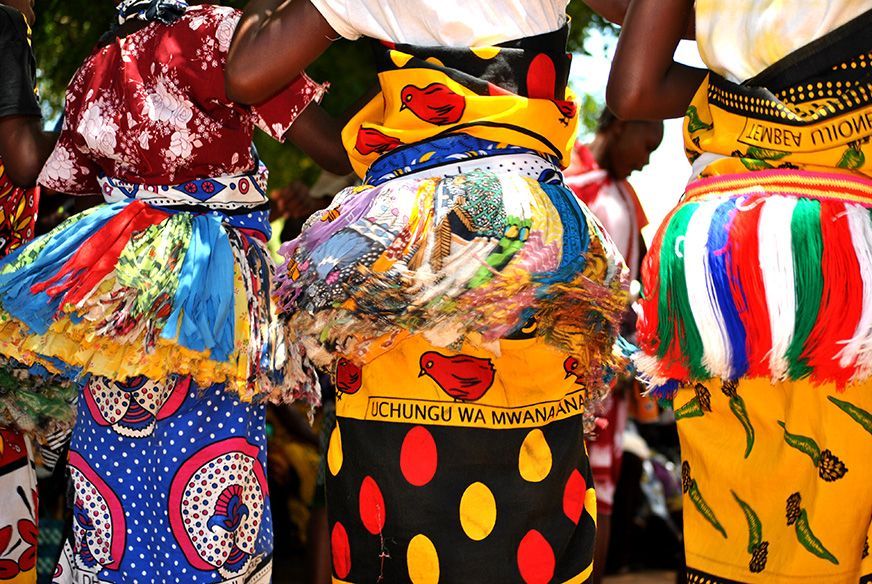This color photograph captures the vibrant rear view of three black women in mid-dance, set against a blurry background of additional dancers. The image extends from their shoulders to their knees, presenting a detailed view of their elaborate and colorful attire. The woman on the left wears a burgundy and white floral blouse paired with a blue, pink, and white polka-dotted skirt, adorned with a shorter, multicolored skirt of hanging fabric strips around her waist. The central woman dons a white blouse with a black skirt embellished with yellow and red polka dots, featuring a bird and the text "Uchanguwa Moana." She also has a scarf wrapped around her waist. The woman on the right sports a white blouse with a bright yellow skirt decorated with plant motifs, and a fringed skirt in red, white, green, and blue hues around her waist. The combination of their dynamic movements and the swinging ribbons tied around their waists enhances the lively atmosphere of the dance.